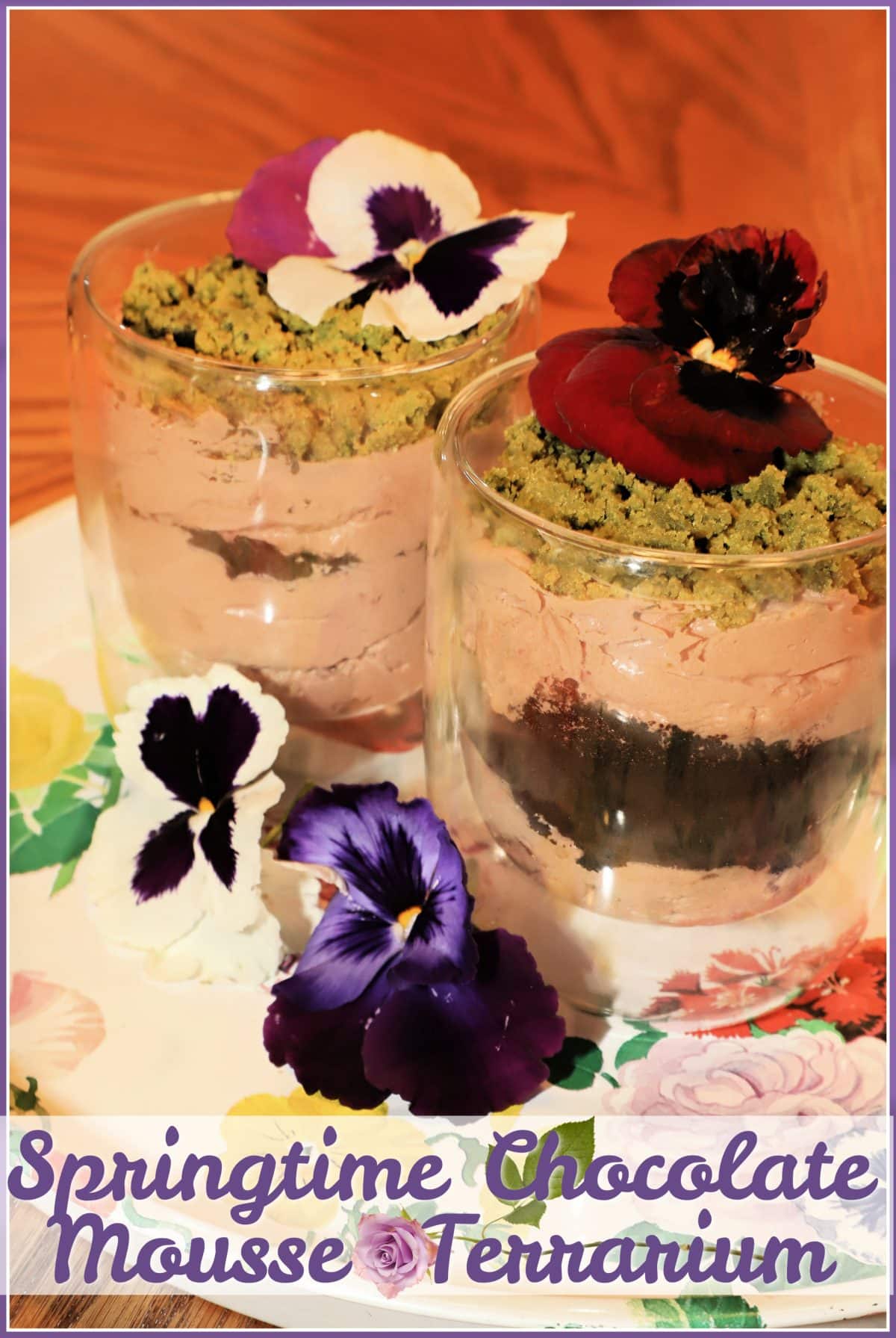The image is an advertisement featuring two glasses of dessert labeled "Springtime Chocolate Mousse Terrarium" in blue cursive at the bottom, set against an orange, wrinkled cloth background. Each glass contains layers of light brown mousse, darker chocolate, and a crumbled cookie-like topping. The dessert is garnished with flowers, including a red pansy with a black and yellow center on one glass, and a white pansy with similar features on the other. In front of the glasses lie additional pansies, one white and one purple, adding an extra touch of springtime elegance. Despite the decorative appearance, the presentation may seem too ornate to be appetizing for some.